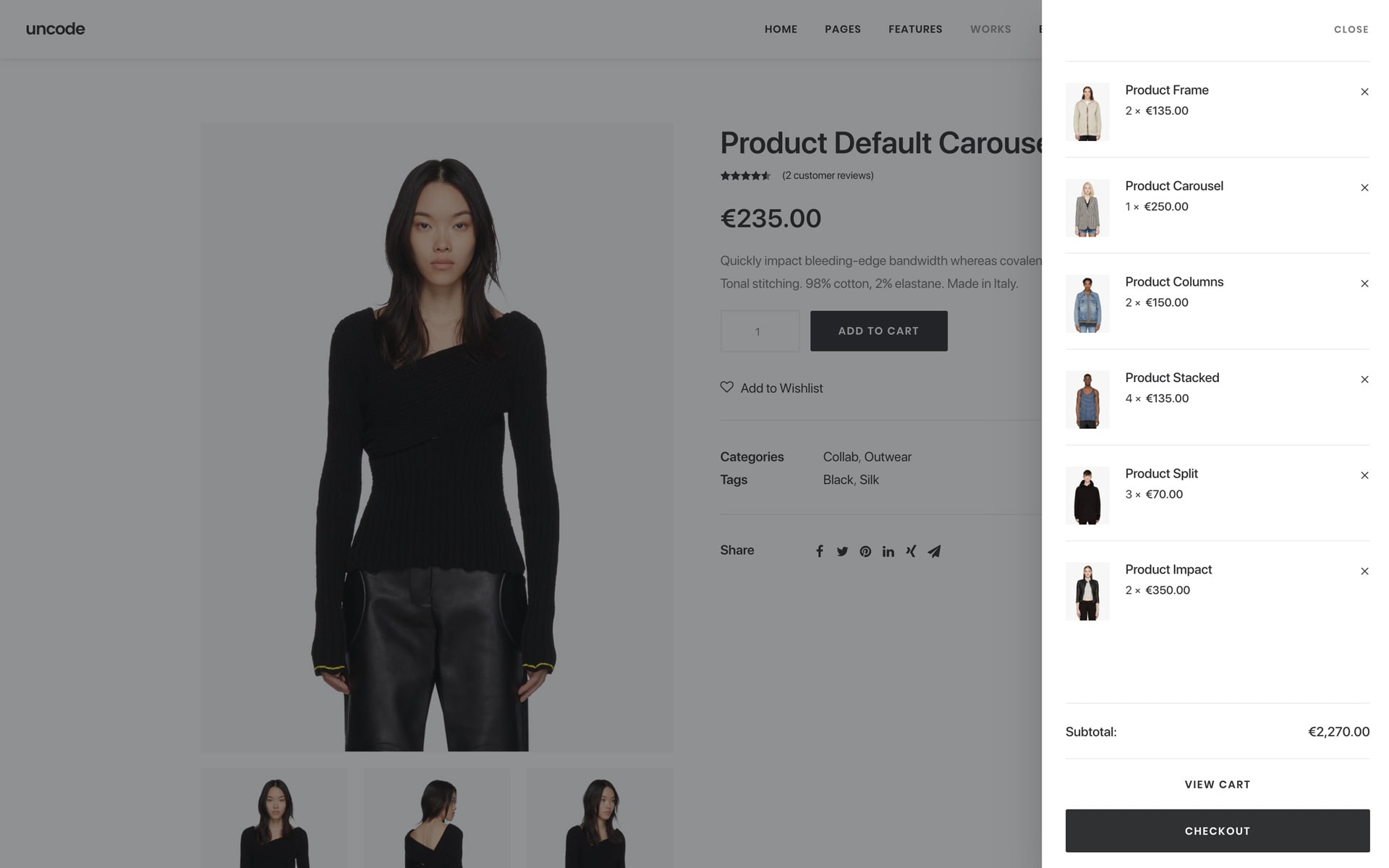A screenshot of an online storefront page showcases a collection of women's clothing against a darkish white or gray background. Central to the image is a darker gray section that features a striking photo of a young, attractive Asian woman. The model, with her straight black hair cut in varying lengths around the ears and chin, appears with a stern expression, gazing directly into the camera. She is dressed in a chic black top characterized by its exceptionally long sleeves that extend past her wrists, nearly covering her fingers. Complementing her top, she wears stylishly baggy pants with a distinctive gray sheen. Positioned to the right of the model at the top of the page is the phrase "Product Default," partially obscured to read "Produc Default Carousel" due to cutoff letters. Directly below, the product boasts an impressive rating of four and a half stars, followed by text too small to decipher entirely, but potentially indicating a promotional event. The final detail includes the pricing information, marked with a British pound sign, listing the item at £235.